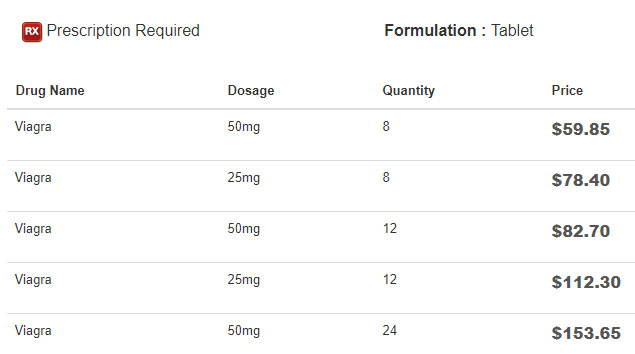This image depicts a detailed chart outlining the prescription requirements for different dosages and quantities of Viagra tablets. At the top of the page, a red square with white letters prominently displays the "Rx" symbol, indicating that a prescription is required for these medications. Below this symbol, a table lists the available dosages and corresponding quantities of Viagra:

- 15 milligrams, quantity: 8
- 25 milligrams, quantity: 8
- 50 milligrams, quantity: 12
- 25 milligrams, quantity: 12
- 15 milligrams, quantity: 24

Interestingly, the prices increase as the quantity and dosage increase, although the 25 milligrams are priced higher than the 50 milligrams, an anomaly that is not explained. The cheapest option listed is the 15 milligrams at a quantity of 8, priced at $59.85. The most expensive option is the 50 milligram tablets in a quantity of 24, priced at $153.65. The entire page is set against a white background with the text in black font, providing clear and easily readable information.